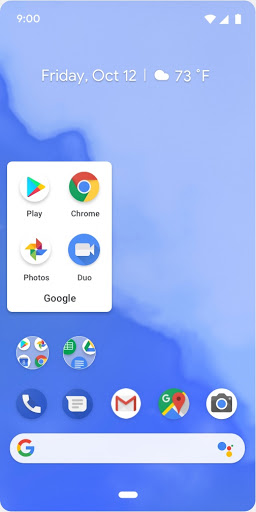The image is a screenshot of a person's home screen on an Android or Google phone. At the top right corner, there are three icons: a fully charged battery icon, a fully filled phone signal strength icon, and a fully filled Wi-Fi signal strength icon, all in white color. On the top left, the time is displayed as 9:00. Centrally positioned at the top, the date reads "Friday, October 12," and to the right of it, there's a cloud icon indicating the weather, with the temperature display reading "73°F."

In the mid-section towards the left, a boxed area with a white background contains four app icons: "Play" in the top left, "Chrome" in the top right, "Photos" in the bottom left, and "Do" in the bottom right. Below this boxed area is a row of seven circular app icons. The bottom row includes icons for Phone, Text, Gmail, Google Maps, and Camera.